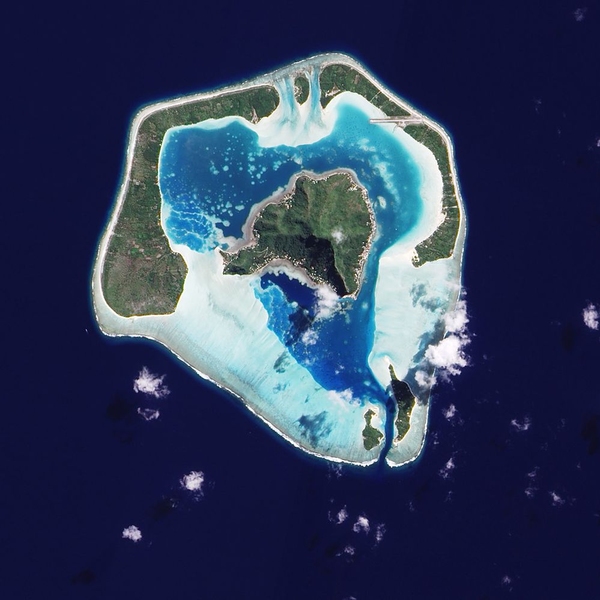This detailed aerial photograph, which could have been taken by a satellite or a high-flying airplane, captures a picturesque group of closely clustered islands. Dominated by rich greenery, the central island stands out with its hilly and mountainous terrain, surrounded by a striking lagoon of light turquoise waters. Encircling this core, smaller islands of varied shapes are set against the deep, dark blue expanse of the ocean. One particularly notable landmass curving and forking to the right adds to the geographical complexity. The islands feature both lush green areas and pristine white sandy beaches, creating a striking contrast in texture and color. The overall shape of the islands collectively forms a rough pentagon with five curved sides, enhancing the stunning visual of a tropical paradise. Wispy clouds are scattered throughout the image, adding an ethereal touch to the vibrant and multifaceted seascape.